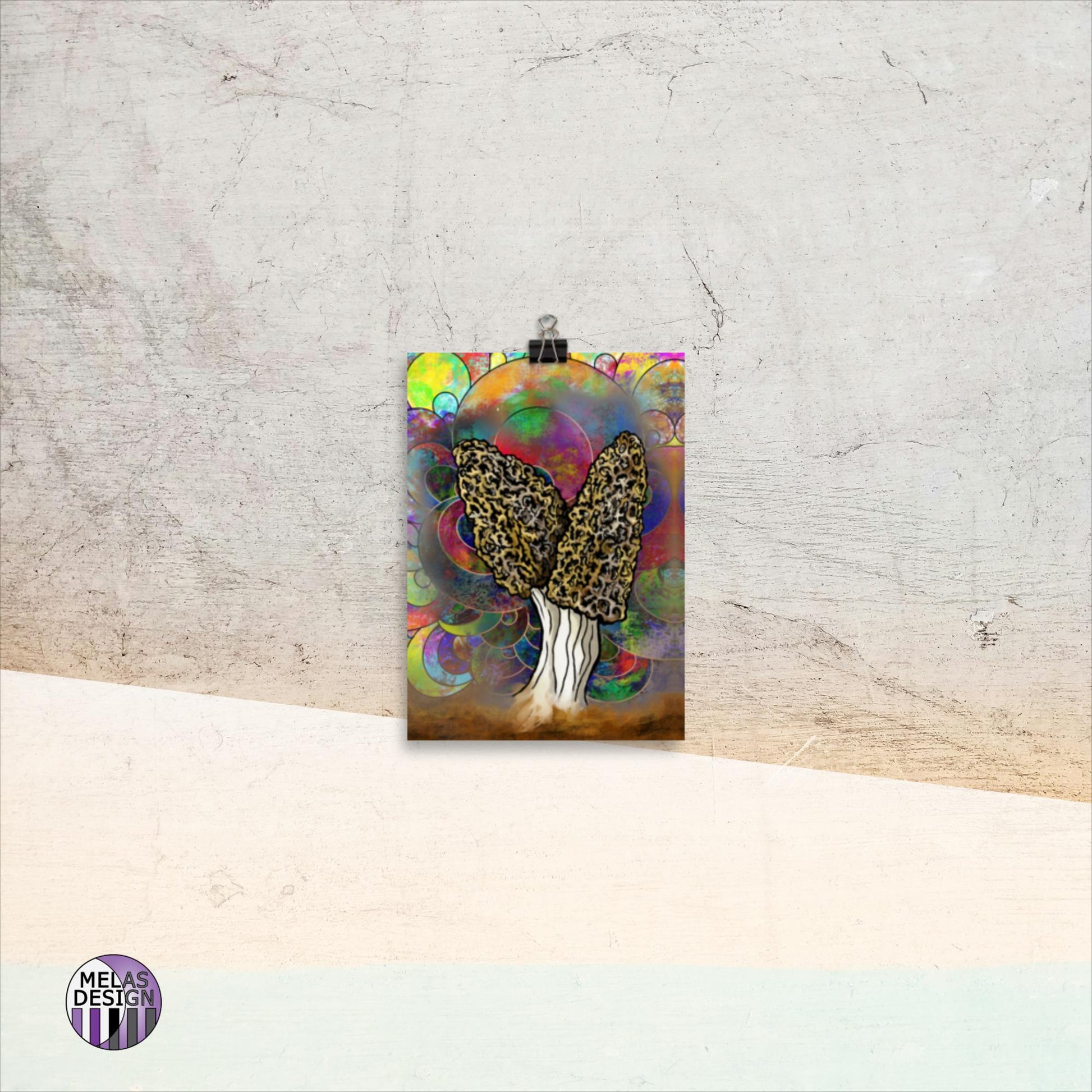The image depicts a clipboard positioned on a white floor against a concrete gray wall, showcasing an artwork of two conjoined mushrooms. The mushrooms, which have white stems and sandy brown, leopard-print-like caps, are graphically illustrated. The background of the artwork bursts with vibrant, kaleidoscopic patterns of interwoven circles and splotches in bright greens, yellows, oranges, reds, purples, blues, and pinks. The entire setting rests against a wall characterized by black lines and cracks, transitioning to a yellowish hue near the floor. At the very bottom left corner of the artwork is a circular logo that reads "Mela's Design" in purple, accompanied by an icon of five tall structures.